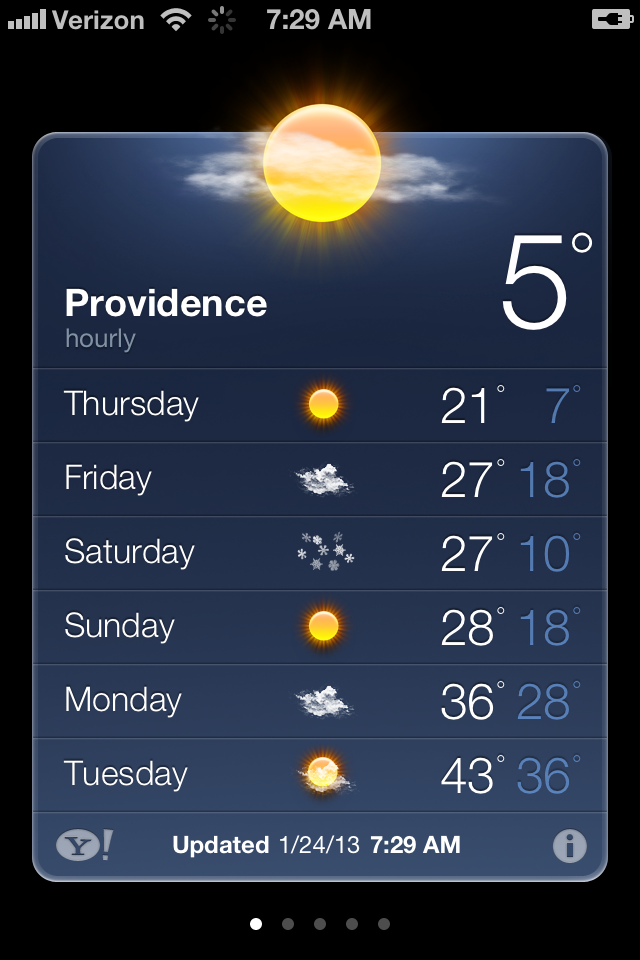This screen capture from a weather app on a cell phone displays a detailed weather forecast for Providence. The interface reveals various status icons at the top: a cell signal indicator, "Verizon," a Wi-Fi signal, a circular icon, "7:29 AM," and a battery icon showing it is plugged in. The background is predominantly black, contrasted by a gradient blue box in the center.

At the top of this blue box is an illustration of a sun partially obscured by clouds, indicating current weather conditions. Below the illustration, the location "Providence" is specified along with the current temperature of 5°C. The segment also indicates that this information pertains specifically to Greater Providence and offers an hourly forecast option.

The forecast spans from Thursday to the following Tuesday. Detailed daily weather icons and temperature highs and lows are listed vertically:

- **Thursday**: A sun icon with temperatures of 21°C (high) and 7°C (low).
- **Friday**: A partially cloudy icon with temperatures of 27°C (high) and 18°C (low).
- **Saturday**: A snowflake icon with temperatures of 27°C (high) and 10°C (low).
- **Sunday**: A sun icon with temperatures of 28°C (high) and 18°C (low).
- **Monday**: A cloud icon with temperatures of 36°C (high) and 28°C (low).
- **Tuesday**: An icon with clouds, indicating partly cloudy conditions, with temperatures of 43°C (high) and 36°C (low).

At the bottom left of the screen, the "Yahoo" logo is present with a time stamp indicating the last update at "1:24.13" on the same date at "7:29 AM." Completing the interface is a gray circle with an eye icon, possibly suggesting more details or settings can be accessed from that button.